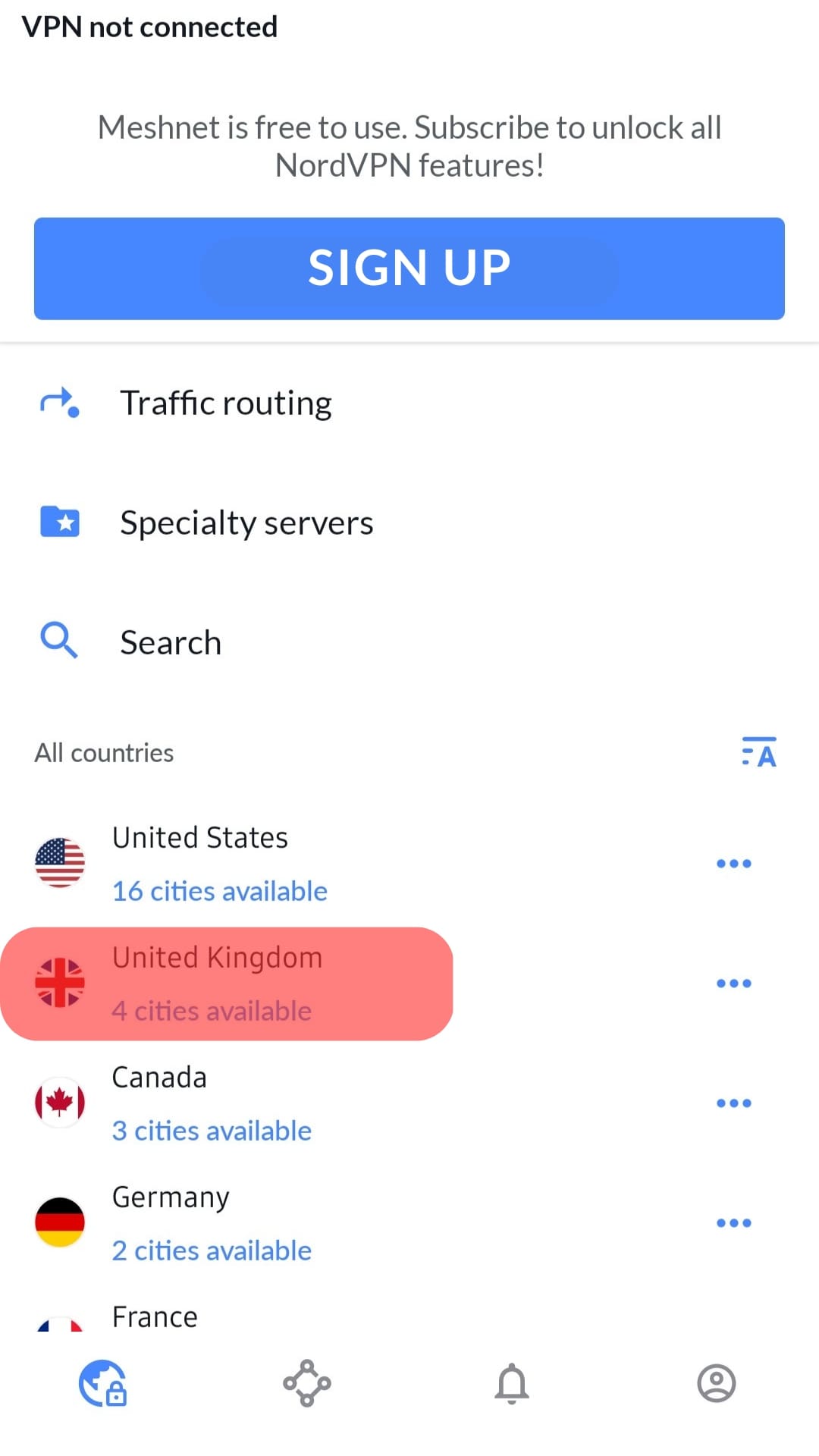The image is a screenshot from a mobile phone, set against a white background. In the upper left corner, bold black text indicates "VPN not connected." Just below, smaller black text reads, "Meshnet is free to use. Subscribe to unlock all the NordVPN features!"

The next section features a prominent purple rectangle with white text in the center that says "Sign Up." A black line separates this area from the content beneath. Directly below the line, a purple arrow points to the right, adjacent to black text that reads "Traffic Routing."

Further down, a purple folder emoji with a white star stands out to the left of the black text, "Specialty Servers." Below that, a purple magnifying glass icon accompanies the word "Searching," which is written in black text. The word "Searching" is positioned to the left of black text that lists countries available for connection: "All Countries," "United States," with "16 cities available" written to the right of a circle featuring a portion of the American flag. 

The text "United Kingdom" follows, placed to the left of a circle with a segment of the UK's flag. This text is highlighted with a translucent red rectangle, and below it, "4 cities available" is noted. Finally, the word "Canada" appears at the bottom of the screenshot.